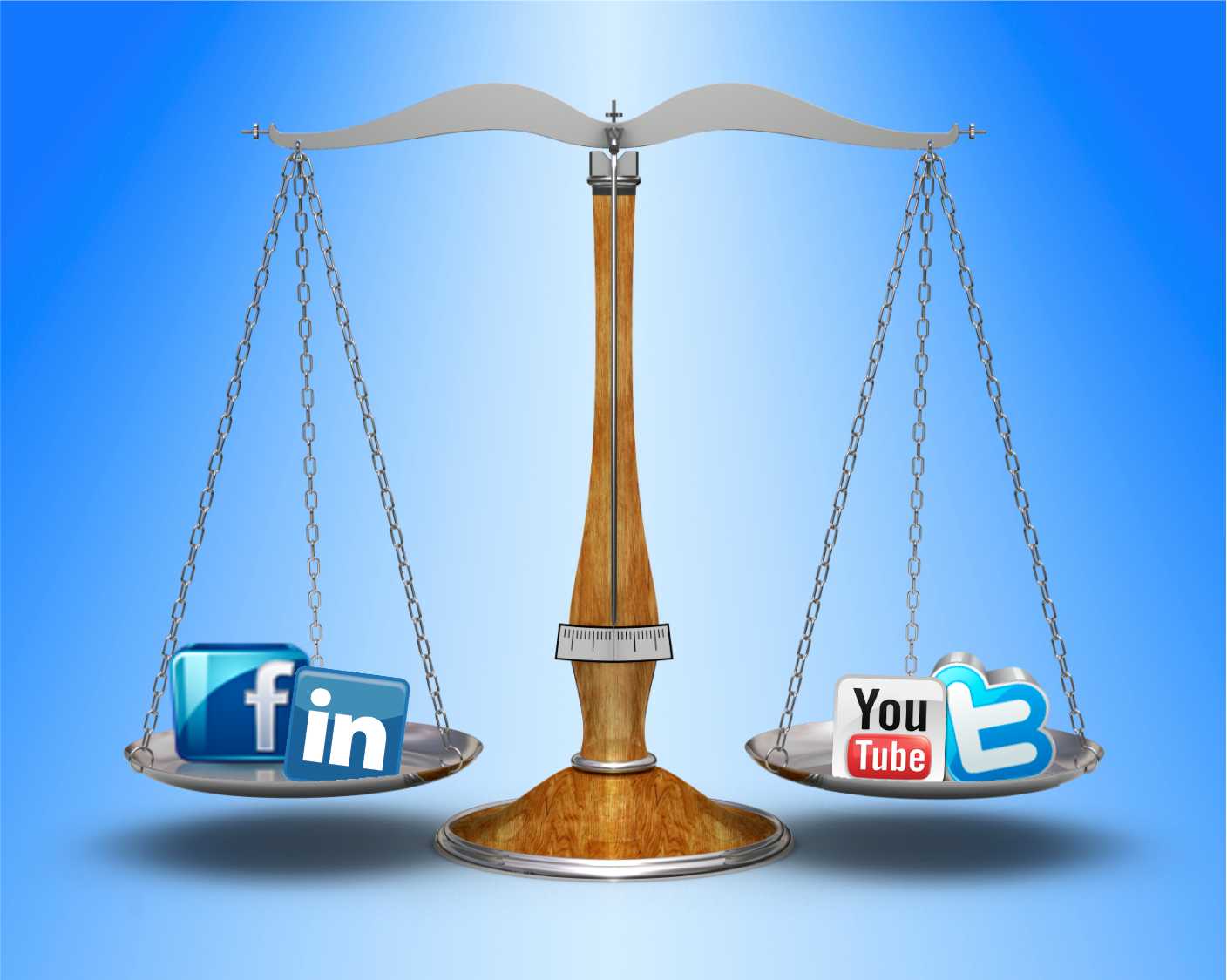The image is a digital illustration of a traditional balance scale, evoking the Scales of Justice, set against a blue background which fades into white under a central spotlight. The vertical base of the scale is constructed from brown wood, adorned with a needle and a slightly curved indicator bar with markings. At the top of the wooden base, a horizontal metal bar extends, supporting two silver dishes hanging by three metal chains on each side. 

On the left dish, there are two social media icons: a glossy blue rounded square with a white lowercase "f" for Facebook, and another square with rounded edges in blue displaying the white text "in" for LinkedIn. The right dish holds two other social media logos: one with a white background and a rounded square showing "YouTube," where "You" is in black and "Tube" is enclosed in a red rectangle; the other is a blue background with a white lowercase "t," symbolizing Twitter, surrounded by a blue outline and silver edges. The scale is depicted as perfectly balanced, symbolizing an equilibrium between the platforms represented.